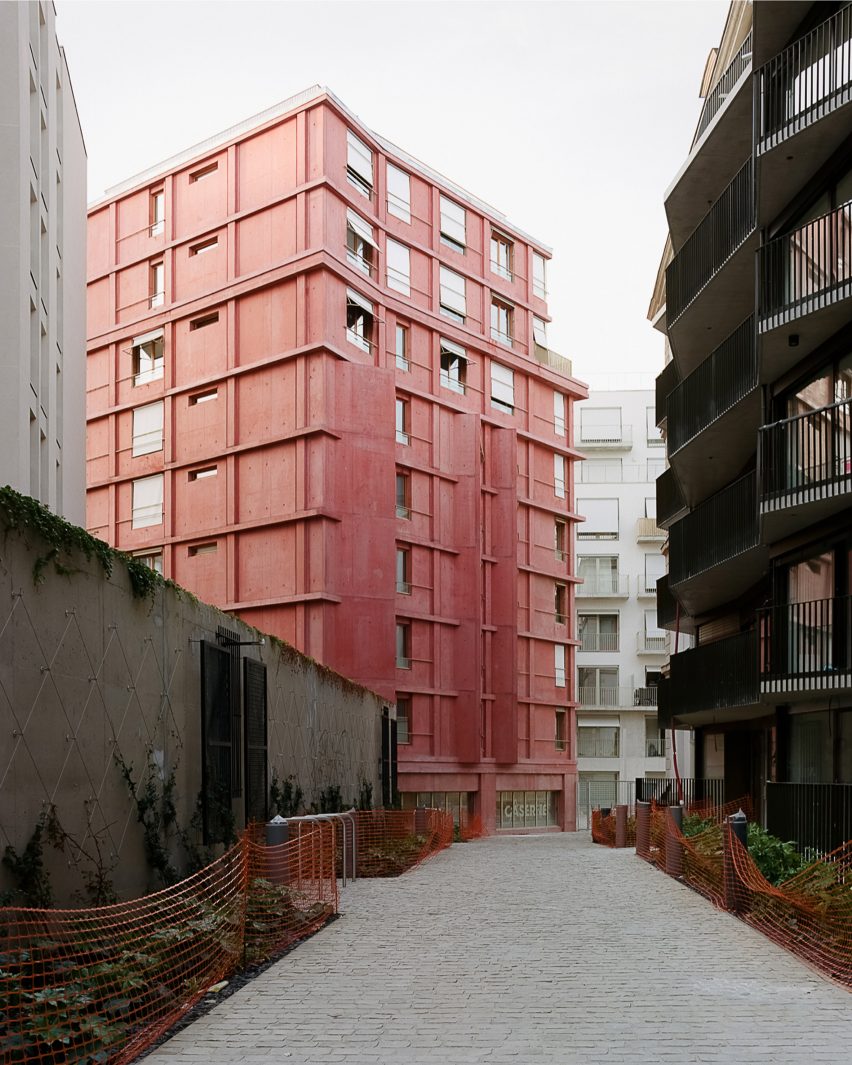The photograph captures an urban scene dominated by a wide, grey brick walkway flanked by a flexible, grid-patterned plastic construction fencing on both sides, standing just a few feet tall. The left side features a single-story grey wall, which leads up to a large red building standing prominently at about 9 to 12 stories tall with a distinctive light red hue. This red structure has a series of rectangular windows, some vertical like those typically found in bathrooms, and others larger and more traditional. 

Directly surrounding this central red building are various other structures indicating a mixed-use residential area. To the right, there's an identifiable apartment complex featuring patios with black railings and sliding glass doors. Further in the background, another tall building, predominantly white, blends into the skyline, creating a layered cityscape with a diversity of architectural styles. The detailed arrangement of buildings and the fenced-off walkway create a vivid portrait of an urban environment in flux, possibly under development.